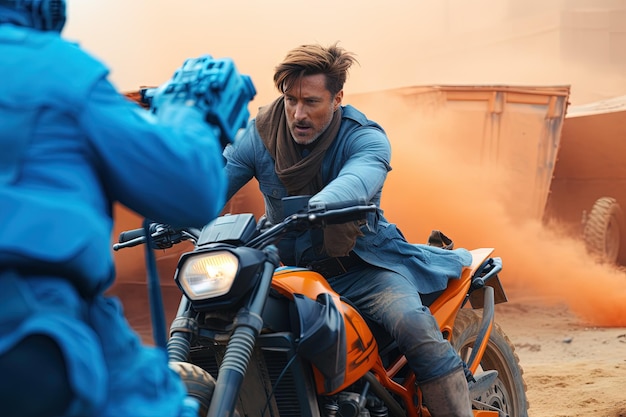In this vibrant still from an action-packed movie, a man dressed in a blue suit and brown boots, with a brown scarf around his neck, is seen riding an orange motorcycle accented with black and blue details. He has short brown hair and a matching mustache, gazing determinedly towards another individual in a light blue outfit who appears to be on a scooter directly in front of him. The scene is set on a sandy terrain, with dramatic orange smoke bombs billowing in the background. An orange spray-painted metal structure stands out among the swirling smoke, and a black tire covered in orange dust is visible in the right corner of the image. The sky, tinged with a smoky orange hue, perfectly complements the dynamism and intensity of the shot.